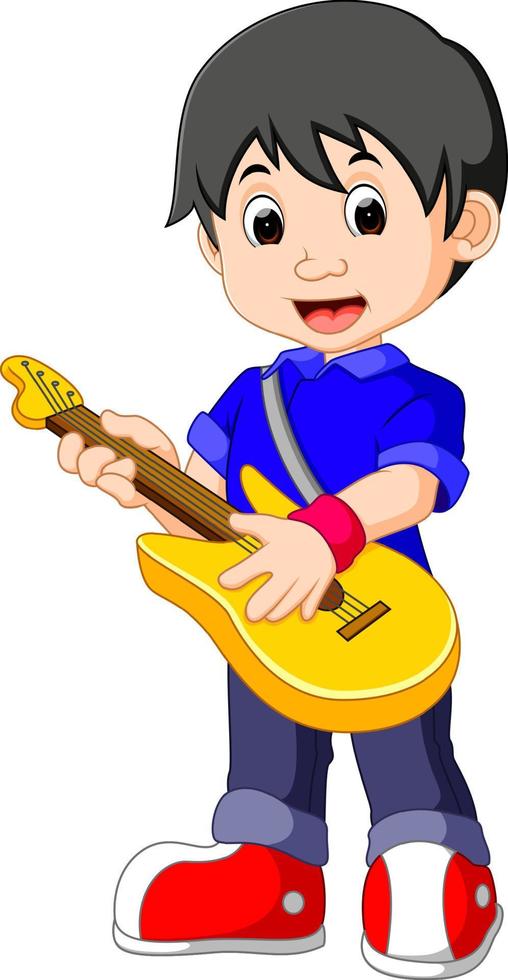This is a digital illustration of a fair-skinned young boy, likely of elementary school age, with dark hair styled in a short cut and dark brown eyes. He is depicted with expressive eyes and raised eyebrows, his mouth open in what seems to be an excited cheer or song. He is dressed in a royal blue shirt, blue jeans that are rolled up slightly at the bottoms, and red and white shoes. Of note is a dark red wristband worn around his arm. The focal point of the image is the boy enthusiastically playing a yellowish-brown electric guitar, with his hand actively strumming the strings and a guitar strap over his shoulder. The background is completely white, putting full emphasis on the boy and his guitar.